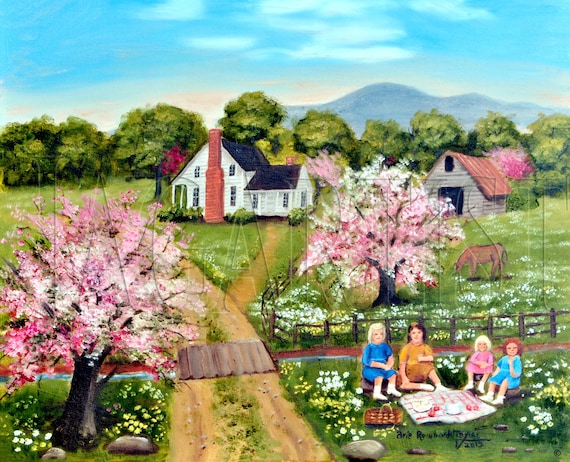This detailed painting depicts a serene country scene centered around a picturesque white farmhouse with a black roof and a prominent brick chimney. Nestled amidst expansive green fields adorned with scattered white and colorful blossoms, the house is approachable via a dirt road that meanders up to its entrance. To the right, a brown wooden fence encloses a lush field. Within this field stands a graceful horse leisurely grazing under the shade of a blossoming cherry tree.

In the background, a small gray barn with a striking red roof and black door adds rustic charm to the landscape which is set against a backdrop of distant mountains beneath a clear, blue sky dotted with fluffy white clouds.

The foreground is vibrant with life, portraying a peaceful picnic on a checkered pink and white blanket, laid out on the grass amid wildflowers and rocks. The picnic is attended by four females, likely a multigenerational family—two women and two children. One woman, possibly a grandmother, has white hair and wears a blue dress, while the presumed mother has brown hair and a yellow-gold dress. The children, around five and ten years old, include a blonde girl in a pink dress and a red-haired girl in a blue dress. Their picnic setup includes white dishes, a basket, and vividly red apples.

The scene is framed by two enchanting cherry blossom trees, one greeting visitors at the entrance on the left and another standing proudly in the field. Nestled in the bottom right corner of the artwork, the artist's signature can be seen subtly inscribed in small black letters, marking the completion of this idyllic countryside tableau.